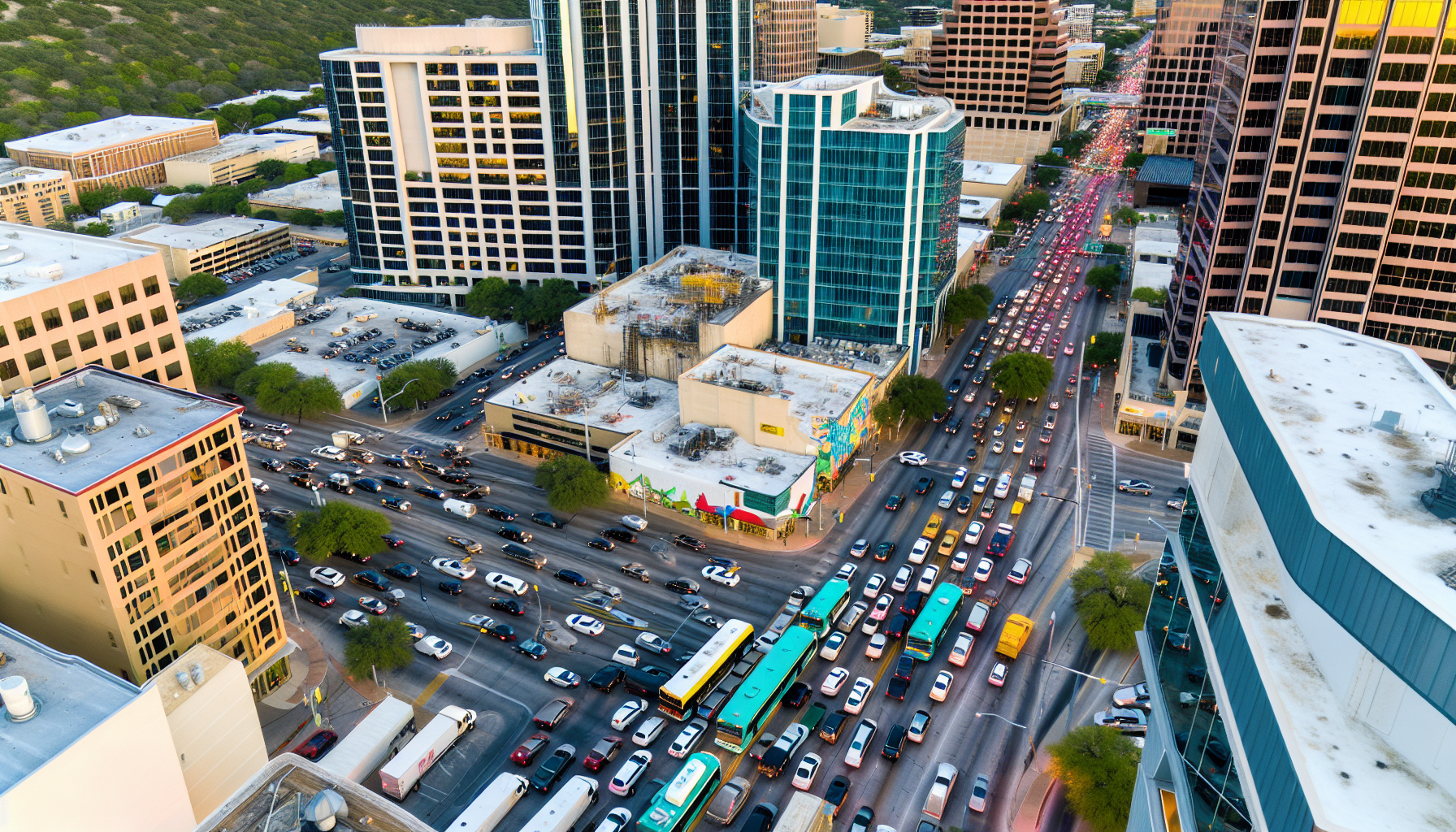This image is a vibrant aerial photograph of a busy city intersection, likely taken from a helicopter or a drone. The scene perfectly captures the hustle and bustle of urban life with a colorful array of vehicles and buildings. Multiple lanes of traffic crisscross in an L-shaped pattern, filled with bumper-to-bumper cars, numerous buses with turquoise and yellow roofs, and clusters of iconic yellow taxis. Skyscrapers and office buildings of diverse shapes and colors—from greenish and brown to white—surround the intersection. The taller buildings reflect the natural sunlight, casting hues of blue and yellow across the glass facades. A few green trees are scattered throughout the urban landscape, offering a touch of nature amidst the concrete jungle. In the distant top left, a hint of green hills suggests a natural backdrop. The rooftops reveal parked cars and air conditioning units, underscoring the industrial aspect of the cityscape. Overall, the photograph is a lively and detailed portrayal of a metropolis in motion.